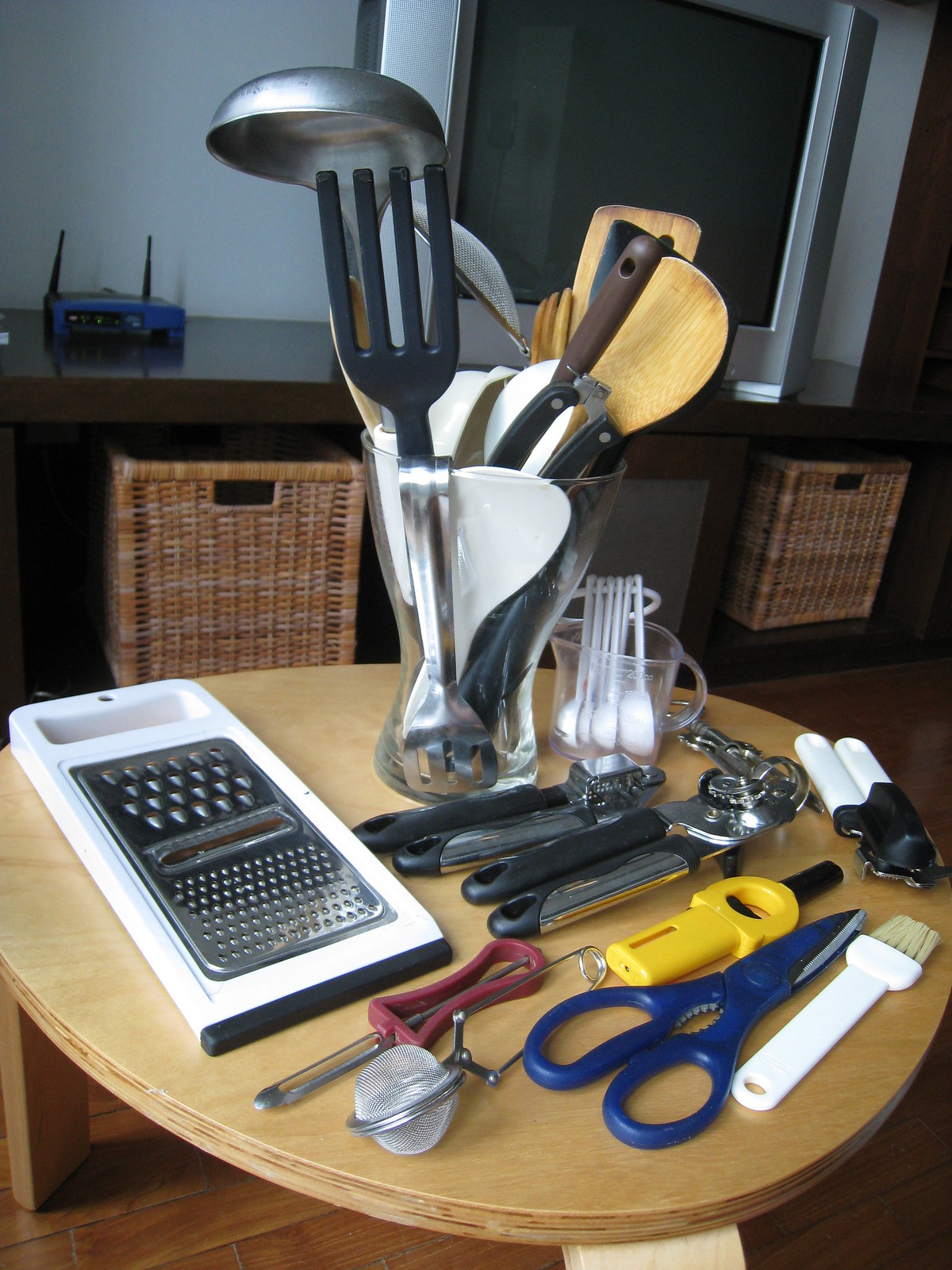The photograph captures a cozy scene inside a home, with the focal point being a small, slightly off-round, modern-shaped, three-legged light wood table. The table is meticulously arranged with various kitchen tools. At the forefront, there is a plastic cheese grater with a metal insert, formed into a tented shape. Nearby lies a potato peeler, a tea ball or strainer, and a pair of kitchen scissors. Next to these is a brush, likely used for basting butter onto dishes like chicken, alongside three manual can openers. Prominently displayed is a set of white plastic measuring spoons nestled within a Pyrex measuring cup. 

Adding to this arrangement, a clear glass vase, which flares at the top, contains an assortment of spoons and forks. Among them are plastic spoons, wooden spoons, a black plastic fork, a wooden fork, and a small strainer. This eclectic mix of utensils is set against the backdrop of a TV stand and television, creating a homely atmosphere. The whole ensemble reflects a practical yet aesthetically pleasing kitchen setup.